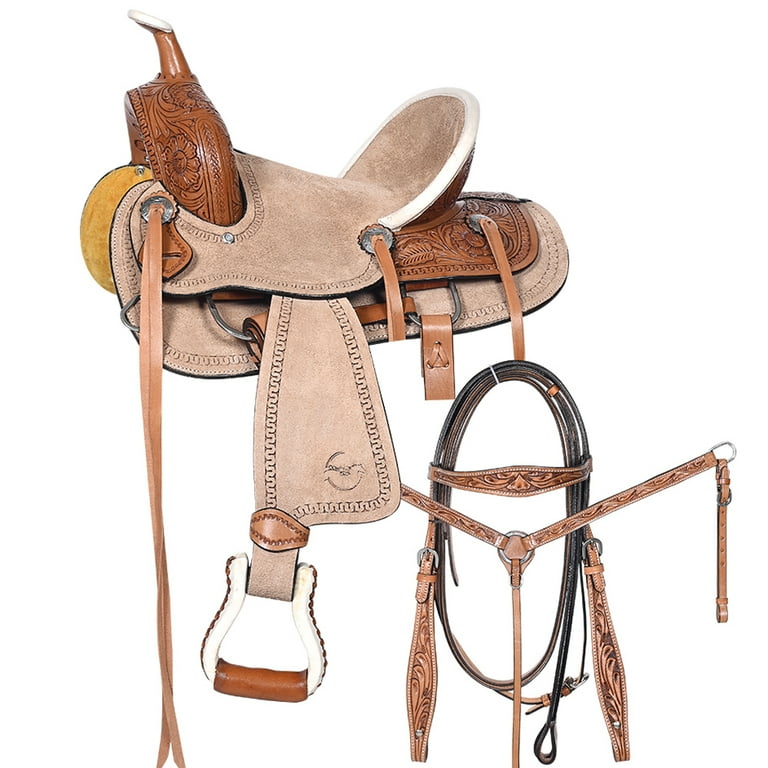This image showcases an intricately designed horse saddle and related riding equipment against a pristine white background. The saddle, characterized by its ornately carved details, combines various shades of brown leather and suede. The main body of the saddle features a medium to dark brown leather embellished with a floral plant design and a lighter brown suede material that transitions into a yellowish hue on the interior. The back of the saddle arcs high, with some sections appearing almost pinkish due to the light. The saddle is adorned with hanging leather strands—some flowing to the ground and others wrapped around the sides. Notably, the stirrups are white with brown leather accents where the foot rests. Complementing the saddle is a harness made from dark brown, detailed leather, and additional straps and ropes are visible, enhancing the elaborate nature of the setup. All these components are depicted as floating in the air, emphasizing the craftsmanship without any background distractions.